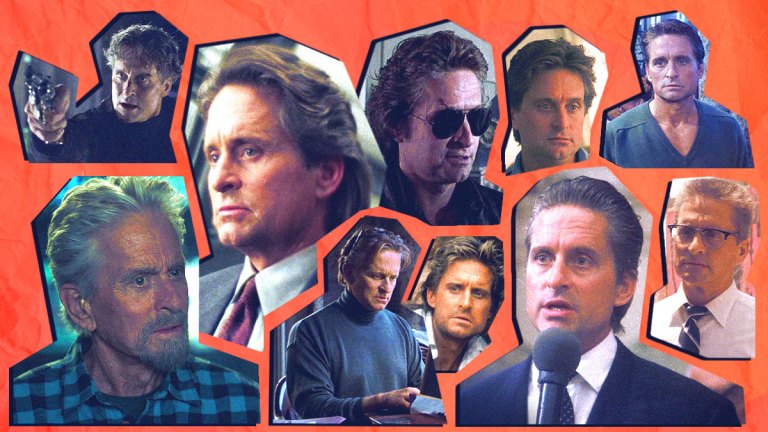The image is a detailed collage consisting of 10 portraits of the renowned actor Michael Douglas, captured at various stages of his illustrious career. Each photograph represents a distinct moment and role from his numerous film appearances, meticulously cut out from magazines or newspapers. The portraits are arranged in an organized manner over a crumpled orange-yellowish background, giving the appearance of being placed on tinted paper. The images feature an array of emotional expressions and outfits: one depicts him with short hair, glasses, a white dress shirt, and tie, looking ahead; another shows him in a suit with a black jacket, white dress shirt, and tie speaking into a microphone. Other notable inclusions are Douglas holding a gun and potentially in roles as a cop, showcasing his versatility and the breadth of his acting career. Each portrait, edged with an approximate 8-10 sided contour, provides a vivid snapshot of Michael Douglas's varied persona through decades of film.